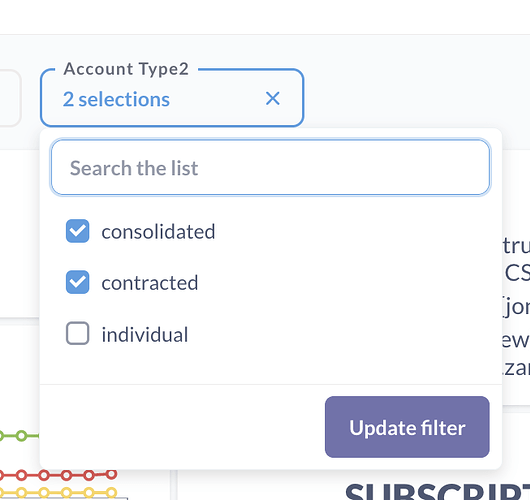A detailed screenshot of a dialog box reveals two selections under the category "Account Type 2" – "Consolidated" and "Contracted," both distinguished with blue checkboxes marked by white checks. Above these options lies a search function for refined filtering. Below the checked selections, an unchecked box labeled "Individual" resides. Positioned to the right of the list, a prominent purple button offers the functionality to update the filter settings.

In the backdrop of the dialog box, partial text is visible through the semi-transparent interface. At the top right, the letters "TRU" are discernible, followed beneath by "CS," then "JO," cut off by the dialog boundary, leaving the succeeding letters partly obscured. Further down, more visible letters include "EW," and even lower, "ZA" alongside the beginning of another letter not entirely legible. At the very bottom, a word that seems to be "subscribed" peeks from the obscured background, offering a fragmented glimpse into the screen behind the active dialog.